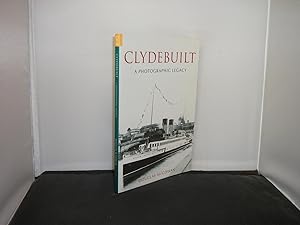This is a professionally taken photograph of a book titled "Clyde Built," which stands vertically on its bottom edge but is tilted slightly to the right. The book is positioned in front of a white shadow box with white walls on either side and is placed on a surface that appears to be black laminate. The book cover features the words "Clyde Built" in bold lettering at the top, with some illegible text below. The central image on the cover is an evocative illustration of a large steamship, reminiscent of the Titanic, with two exhaust stacks, possibly situated in a harbor or at port. The book’s spine is green with some yellow at the top. The white cover of the book stands out against the dark surface, and the overall setup suggests that the photograph aims to showcase the book in a clear and professional manner.